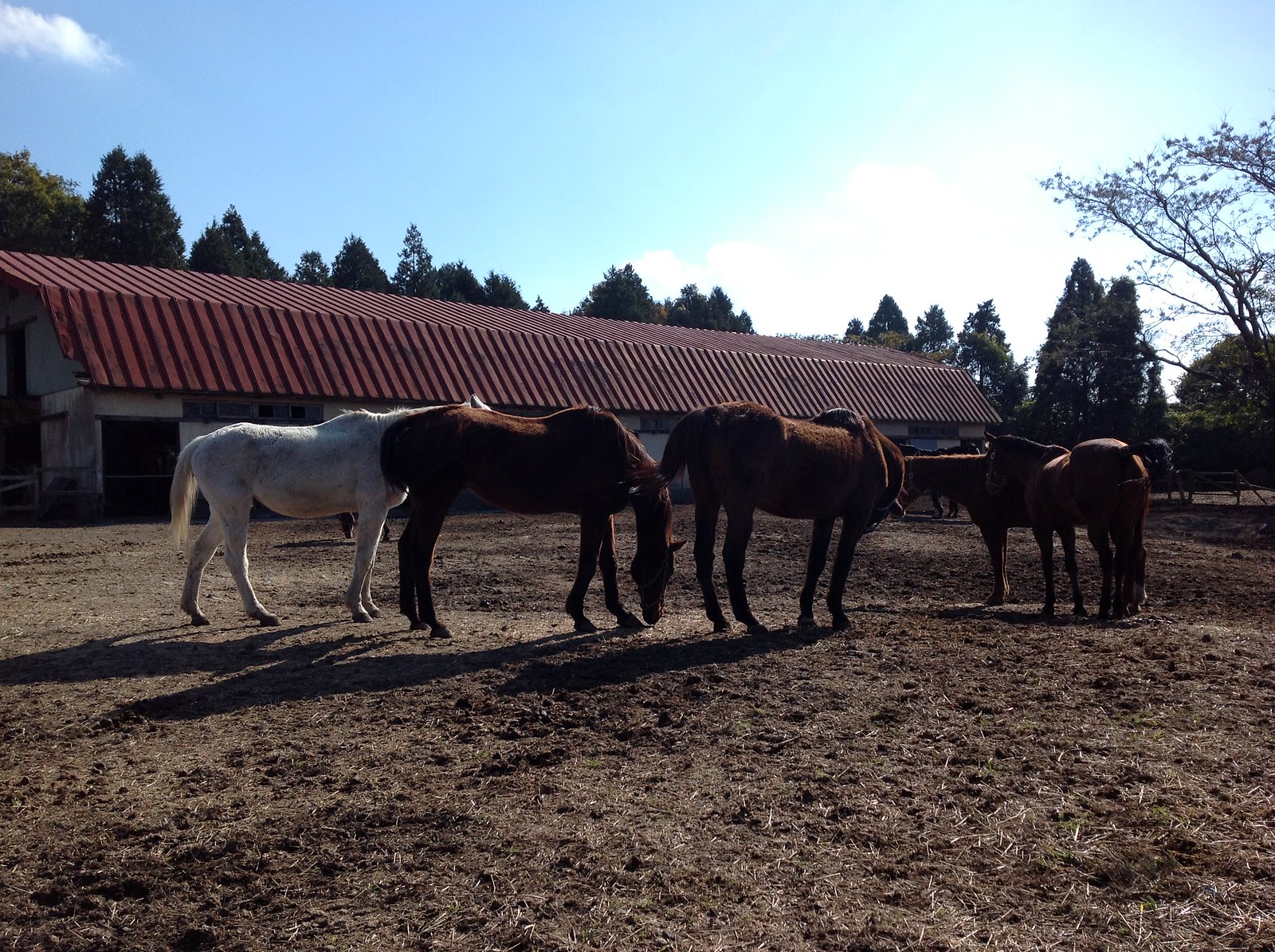The image displays a group of five horses in a dirt-filled enclosure at a ranch, with a rugged patch of scattered hay and sparse, dry grass underfoot. The majority of the horses are a dark chestnut brown, while one is distinctly white, positioned on the left side of the photograph. The animals appear young and healthy, with some casting noticeable dark shadows on the ground. They are either facing away or oriented sideways, partially obscured by one another.

In the background stands a long, white stable or barn with a red roof that slopes down over the sides. The roof features distinct slats across its surface. The right side of the image reveals a bare, spindly tree, while other trees with more leaves and some green bushes continue along the horizon, framing the scene. The sky above is mostly clear with a bright blue hue, save for a single cloud in the upper left corner. The sunlight appears intense on the right side, suggesting either sunrise or sunset.